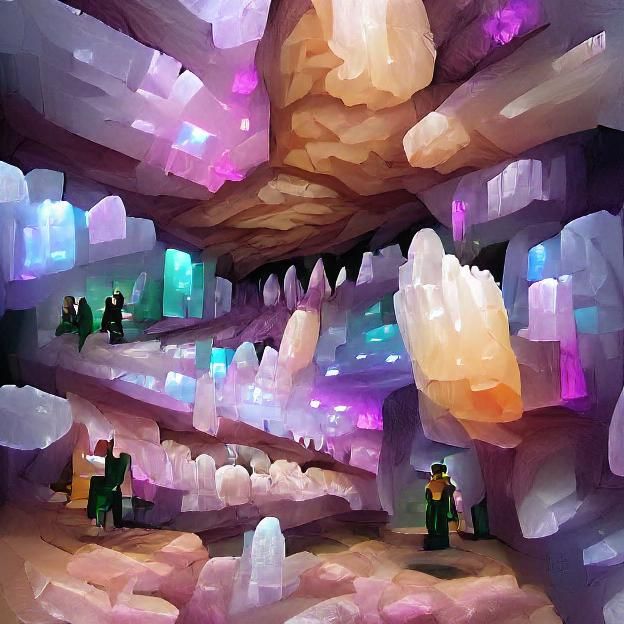This square painting, measuring approximately four to five inches on each side, presents an abstract depiction of an intricate cave environment, reminiscent of a cavern or even an interior space like a shopping mall built within a cave. The cavern is adorned with a captivating array of crystals and quartz, painting the scene with hues of pinks, purples, blues, orange, and a hint of peach. The cave walls and ceiling, predominantly light purple, pink, beige, and brown, are intricately detailed, suggesting natural rock formations with both stalagmites and stalactites prominent in the composition.

At the top center of the image, the cave's brown ceiling anchors the scene, while the left side showcases large pink crystals juxtaposed with smaller, slightly more orange-hued crystals on the right. The center extends down into deeper shadows of black, suggesting the cavern’s depth. The crystals cascade down at a sloped slant, creating the illusion of a walkway. Along this path, abstract impressions of people in green robes emerge; these figures lack distinct features, blending into the scene with hints of greens and yellows.

One of the most striking features is a ramp that inclines from the center toward the left edge of the painting. Some figures appear to be positioned along this ramp, particularly toward its top-left end. Additionally, a figure adorned in green stands out at the bottom right of the image, seemingly in front of an arched doorway, reinforcing the enigmatic cave scenario. The overall scene is richly detailed and complex, inviting viewers into an otherworldly cave-like space bustling with abstract human activity.